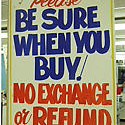This up-close image captures a white sign with a vibrant yellow border, prominently displayed in a store. At the top of the sign, the word "please" is written in cursive with red ink. The center of the sign features large, bold text that firmly states, "be sure when you buy," accentuated by a slim exclamation point. Below this message, in large, bold red letters, is the warning, "NO EXCHANGE OR REFUND," with the word "or" rendered in cursive. In the background, the store is illuminated by overhead fluorescent lighting. A shelf displaying various items, including some dark-colored and red objects, can be seen, while a light blue item is visible on the left side of the image. The top and bottom edges of the sign are slightly cut off, adding a candid, in-the-moment feel to the photograph.